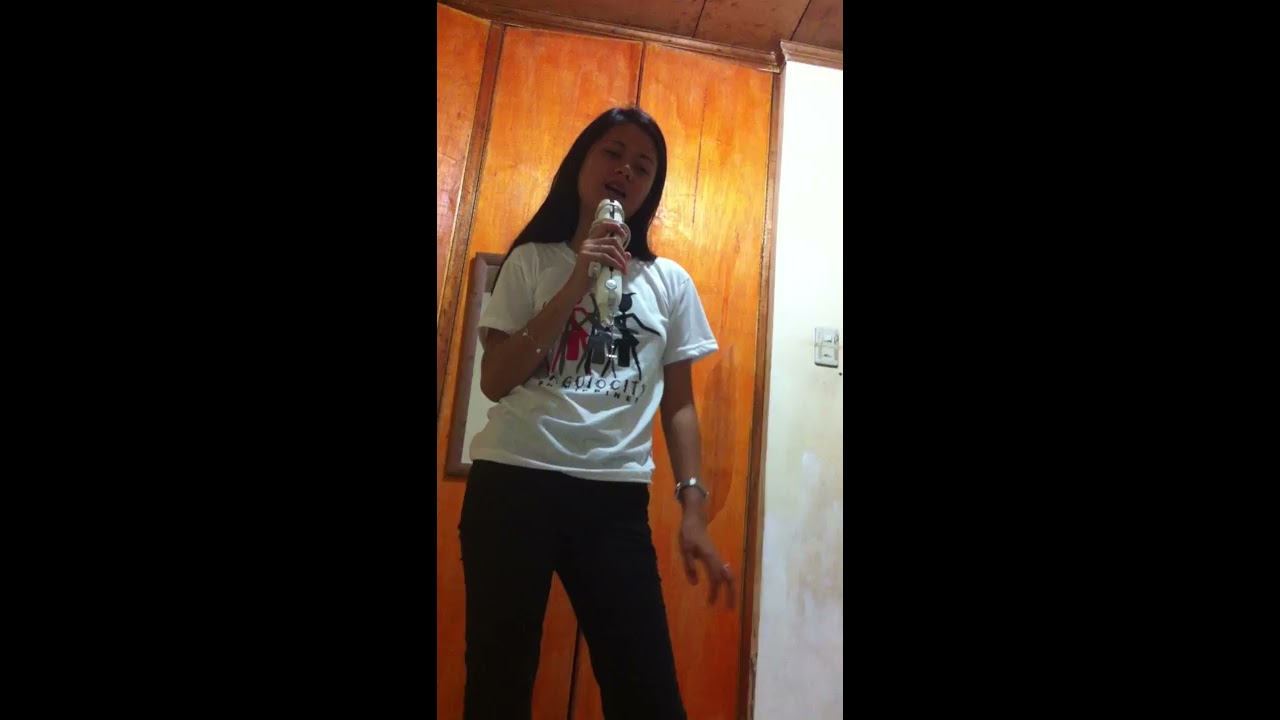The image depicts a young, teenage girl with long, straight black hair, wearing a loose-fitting white short-sleeve shirt adorned with a difficult-to-discern logo or colorful design featuring black, gray, pink, red, and blue elements. She pairs it with average-fit black pants. On her right wrist, she wears a watch, and she has a bracelet on each wrist, as well as a ring on one of her fingers. In her left hand, she holds a white microphone close to her mouth, suggesting she is either singing or speaking into it with great enthusiasm, possibly engaged in a singing video game. She stands in front of a distinctive backdrop featuring a brown wood-paneled wall on the left side and a white wall with a light switch towards the middle, and she appears to be looking down, perhaps reading lyrics or words. The composition includes very thick black borders on both the left and right sides, each as wide as the central image itself.